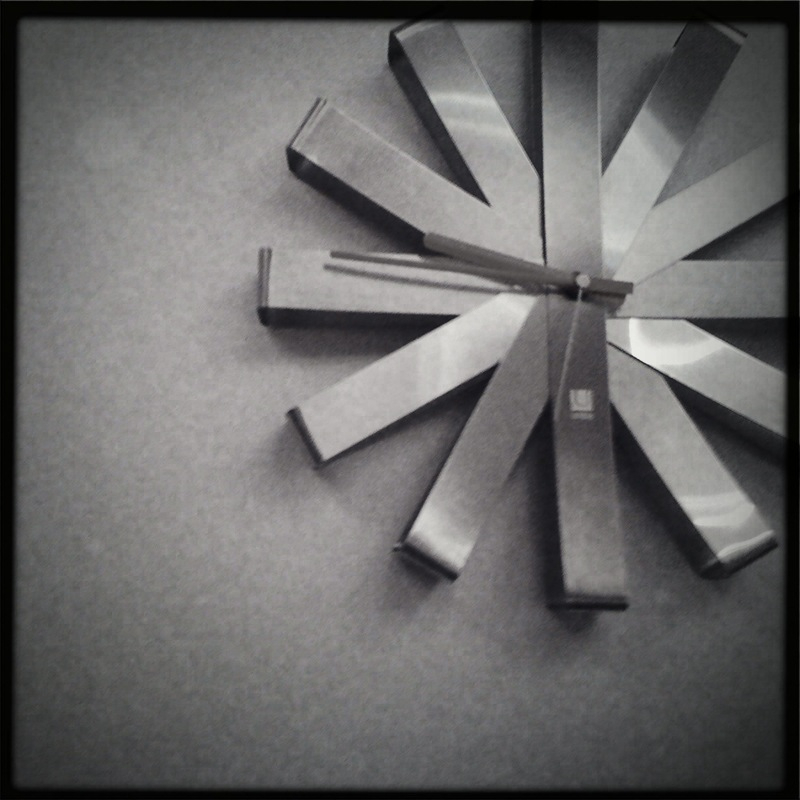This black and white photograph captures a large, abstract, metal wall clock affixed to a wall in the upper right corner of the image. The design is reminiscent of a starburst or sunburst, constructed from rectangular strips of stainless steel arranged in a circular pattern, each pointing to where the hours would traditionally be marked. Each metal strip likely represents an hour, from 1 to 12, creating an almost asterisk-like appearance. The clock's hands are prominent, with darker hour and minute hands and a lighter second hand, and the time appears to be approximately 9:45 to 10:00 p.m. At the center of the clock, there is an indistinct logo, a white square potentially featuring a "U", though the brand name is unclear. The wall behind the clock is gray and splotchy, adding to the monochromatic ambiance of the photo. The overall image has a dark, filtered look with an ombre shadow effect, emphasizing the clock's stainless steel materials and unique design.